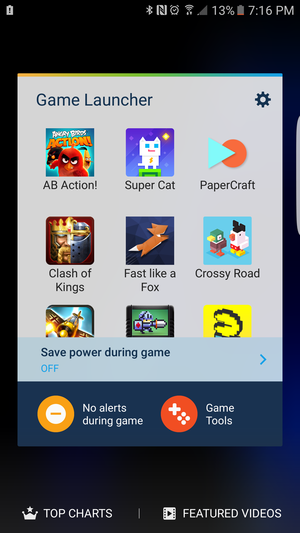Screenshot of a mobile phone display at 7:16 PM with a battery level at 13% and one bar of network signal. Various icons are present at the top-left corner. The image has a black background gradient fading to dark blue toward the bottom-right corner. In the center, a gray box titled "Game Launcher" is visible, featuring a settings icon. Within this box is a list of games arranged in a grid: "AB Action" at the top-left, followed by "Super Cat" and "Paper Craft" to its right. The second row includes "Clash of Kings" on the far left, "Fast Like a Fox" in the middle, and "Crossy Road" on the far right. Beneath the games list, there is a box labeled "Save Power During Game," which is turned off. Below this, another dark gray box displays options for "No Alerts During Game" and "Game Tools."